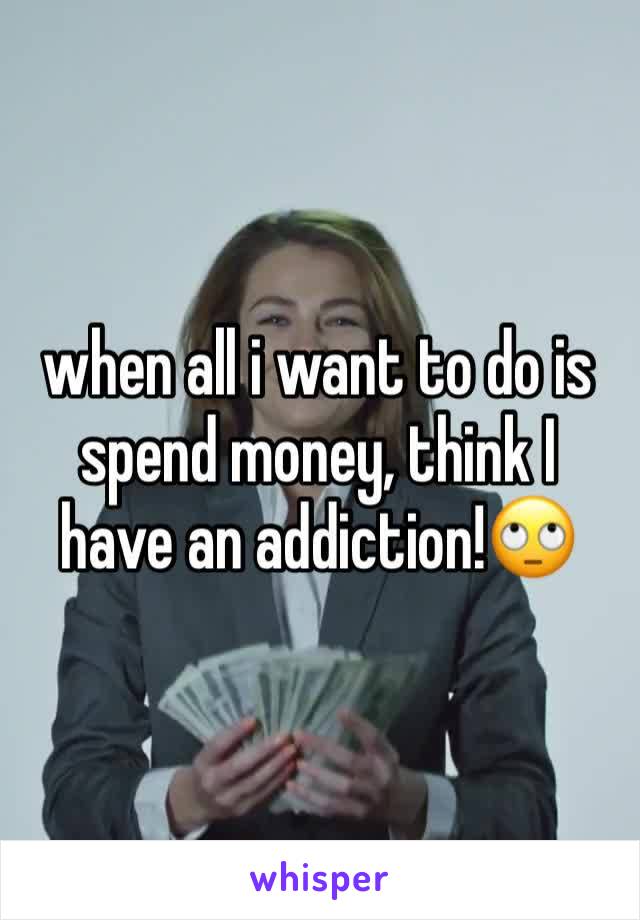The image appears to be a meme featuring a woman dressed in a gray suit jacket over a white shirt, smiling as she holds a fanned-out stack of money in her hands. The woman has light brown hair with blonde streaks and light-colored eyes. Her nails have a polished look, possibly in orange or light pink. The background is a plain gray, likely a wall. Overlaid on the image is white text with a black outline, reading: "When all I want to do is spend money, think I have an addiction," accompanied by an eye-rolling emoji. Below this text, at the bottom of the image, is the word "whisper" in all lowercase letters, presented in bright purple font over a white background. A light source above her head highlights the top of her hair. The overall setting suggests she could be at home or in a store, ready to spend some money.